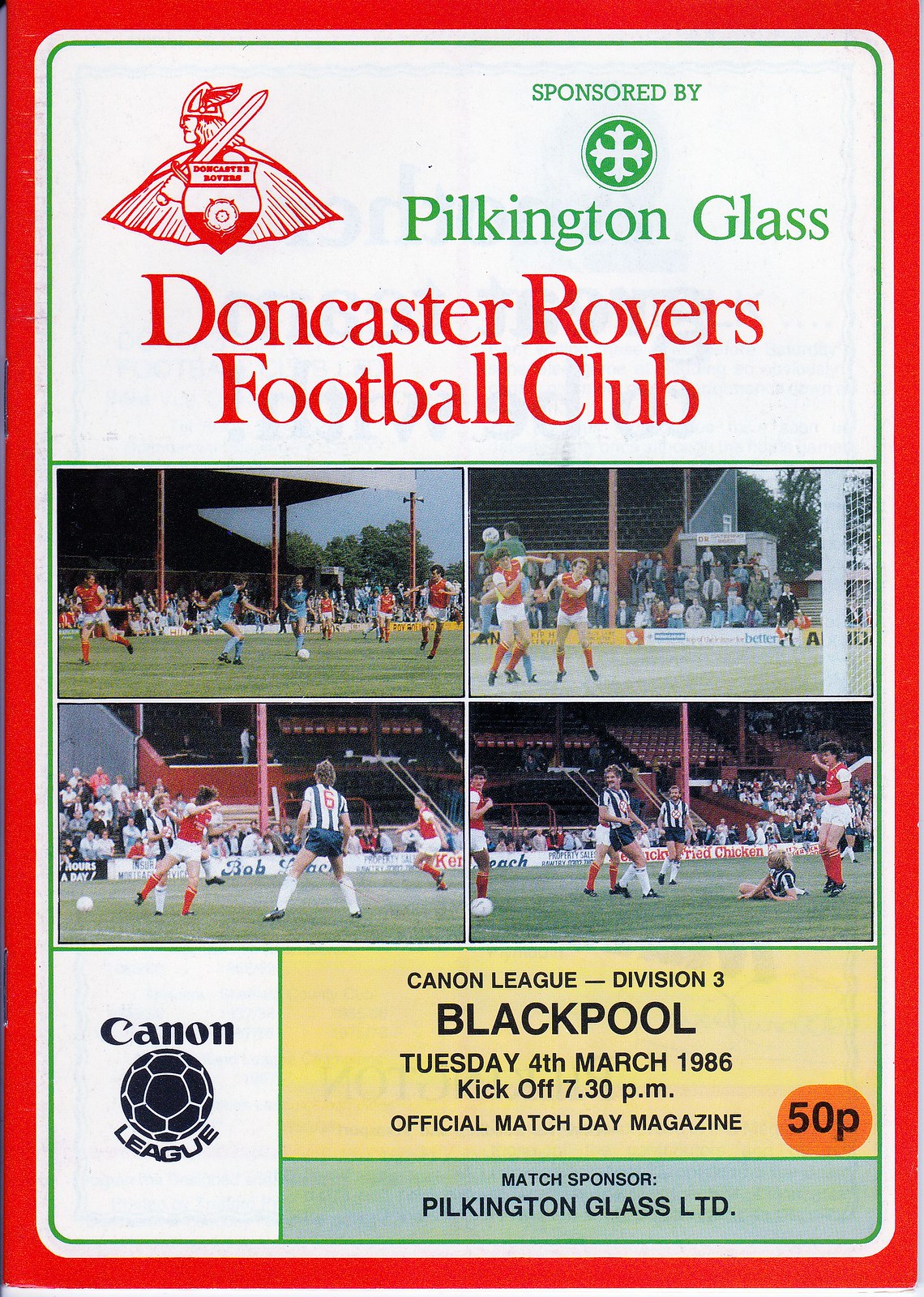The image is a detailed cover of a football game program. It features a prominent red border with a white background. At the very top, in a green font, it reads "Sponsored by Pilkington Glass" with the Pilkington Glass logo, which is a round circle with a white cross. Below this and to the left is a Viking logo representing the Doncaster Rovers Football Club. Beneath these logos, larger red text states, "Doncaster Rovers Football Club." 

The main section features four evenly-sized pictures arranged in a grid, showcasing Doncaster Rovers players in red shirts, white trunks, and red socks in action during matches. Spectators can be seen in the background of each image.

At the lower section of the cover, there is a black and white soccer ball graphic next to the text "Canon League" on a white background. To the right, on a tan background with black lettering, it reads "Canon League Division III Blackpool, Tuesday, 4th March 1986, kickoff 7.30 pm, Official Match Day Magazine." In the lower right corner, on a small blue background, it mentions "Match sponsor: Pilkington Glass Limited." The magazine is priced at 50 pence.